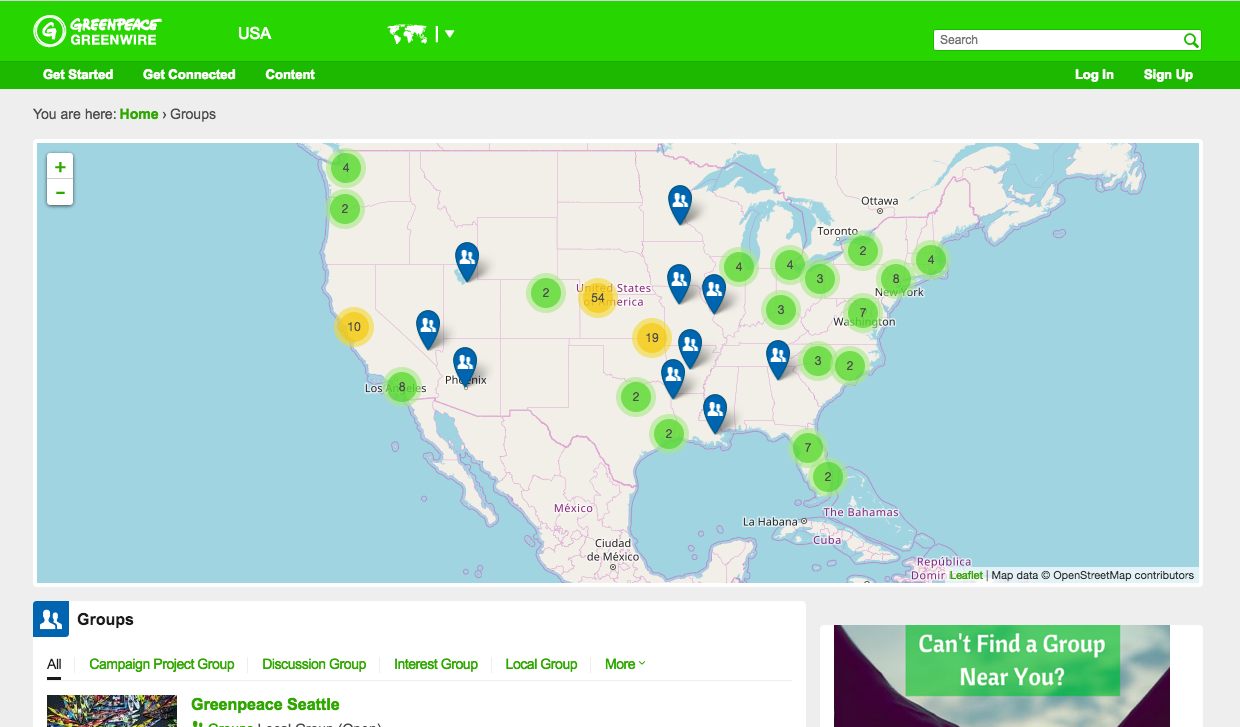The image displays an interactive interface, presumably for a company's internal or customer-facing platform, with several key elements. At the top, there is a long, green rectangular search bar area. To its left, text reads "Green Piece, Green Wire," possibly indicating the company's name or a specific section of the interface. To the right of the search bar, the abbreviation "USA" is displayed alongside an outline map of the United States in white. The search bar itself is active, complete with a magnifying glass icon on the far right for initiating searches.

Beneath the top search bar area, there are clickable options labeled "Get Started," "Get Connected," and "Content." The breadcrumb navigation shows "You are here: Home," with "Home" highlighted in green, followed by an option for "Groups."

The main section of the image features a detailed map of the United States. The map is populated with various markers: green circles displaying numbers, teardrop-shaped icons containing silhouettes of heads, and three yellow circles with the numbers 10, 54, and 19 inside them. Below the map, there is text that reads "Groups: Green Piece Seattle." To the right of this, there is an interactive clickable text saying, "Can't find a group near you?"

This caption provides a thorough description of the interface's layout and functionalities, giving a clear understanding of its purpose and usability features.